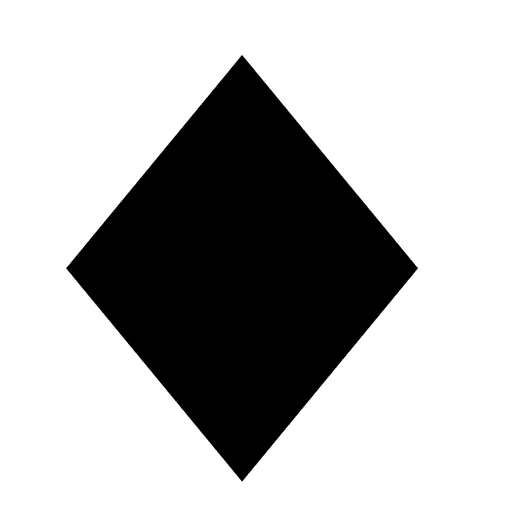The image displays a simple, 2D black diamond set against a plain white background. The diamond is positioned upright on one of its points, creating a symmetric appearance with one point facing upwards, one downwards, one to the left, and one to the right. The diamond appears slightly taller than it is wide, approximately three inches tall and two and a half inches wide, emphasizing a vertical orientation. The shape is reminiscent of two equal triangles joined together, resembling a playing card symbol or the silhouette of a mountain with its reflection. The black color of the diamond is consistent and solid, with no gradients or variations. The image has been created digitally, without any text, additional colors, or context surrounding the diamond.